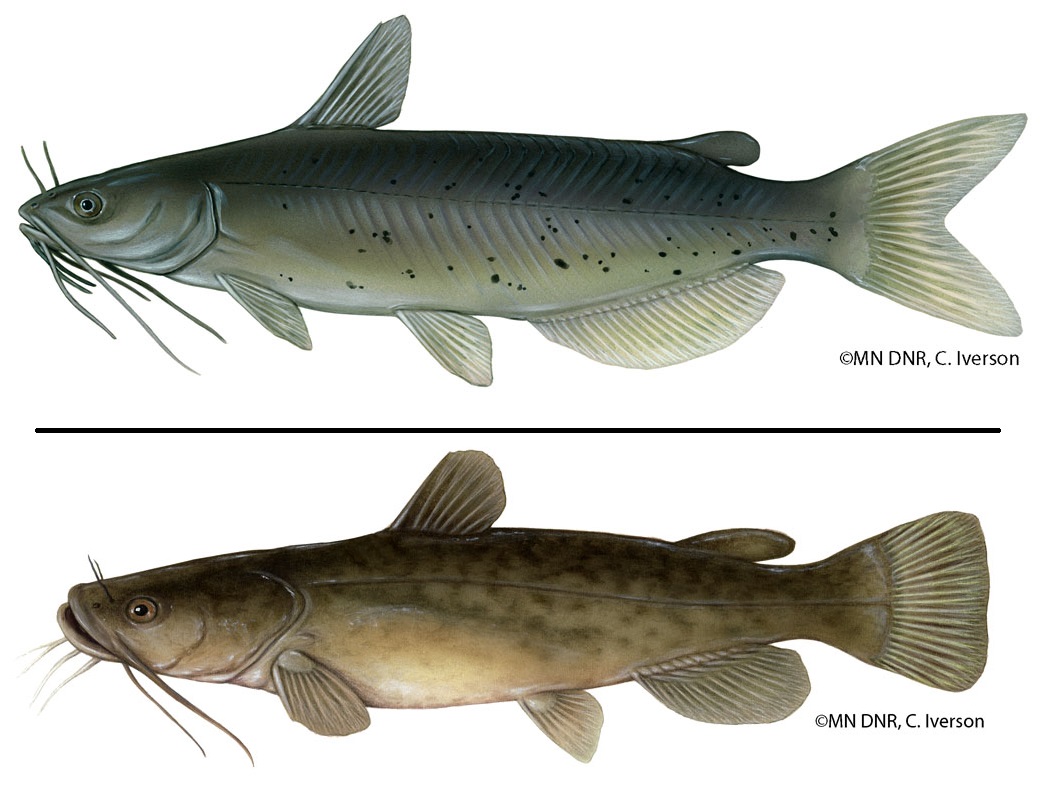The image collage consists of two distinct fish illustrations, separated by a black line. Both fish are oriented with their mouths and eyes facing towards the left, showcasing similarities with subtle differences in their appearances.

The top fish displays a bluish-gray coloration adorned with black speckles scattered across its scales. Noteworthy features include several antenna-like appendages hanging from its mouth and two additional antenna-like structures above the eyes. The dorsal (top) fin is prominently displayed, and the fish is equipped with three ventral (bottom) fins: one located at the front, another positioned mid-body, and a final fin towards the rear, ending with a typical fish tail.

In contrast, the bottom fish exhibits a brownish-tan hue with blue speckles. This fish mirrors the top one in its fin arrangement, with three ventral fins and a dorsal fin, as well as similar antenna-like features extending from the mouth and the lower body. The additional hairs or appendages around its mouth give it a distinct appearance.

Both fish illustrations bear the copyright notice "© MN DNR, C. Iverson," indicating their origin and licensing.